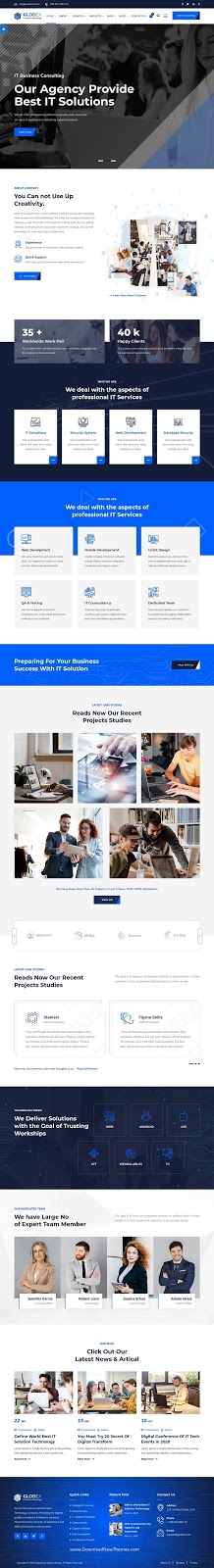**Descriptive Caption for an IT Solutions Business Web Page:**

The web page is a professional business site dedicated to providing top-notch IT solutions. The overall color scheme is a clean and corporate blue and white. At the top, there's a headline emphasizing the agency's commitment to delivering the best IT solutions. Despite the low resolution making details hard to discern, there are clear sections featuring testimonials and showcased statistics, possibly indicating client satisfaction and company performance metrics.

Prominently featured is the "About Us" section, which highlights the company's inclusive culture with images showing a diverse team of two women and two men designated as expert team members. The site aims to build trust through workshops and other interactive services, although some of the text appears too dense and cluttered, contributing to a less than optimal user experience.

At the bottom of the page, a blue bar contains legal disclaimers and menu options for further navigation. There's also a notable emphasis on creativity within the IT solutions realm, even though some of the elements appear too packed into the available space, making specific details difficult to read due to the resolution issue. Overall, it embodies the aesthetic and functional elements typical of a modern IT solutions business website.